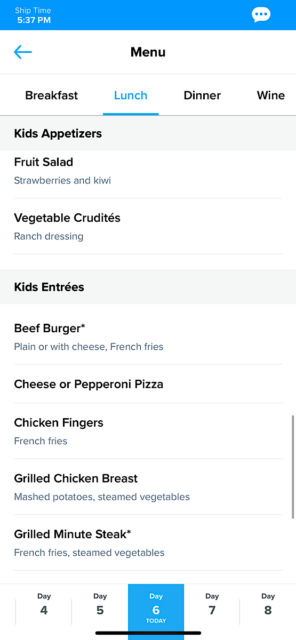The image depicts a digital menu interface, likely on a device resembling an iPad or iPhone, characterized by its tall rectangular shape. A blue strip spans the top of the screen, displaying "ship time, 5:37 PM" in a crisp white font. Below this, a dialogue box with three dots, designed to resemble a chat window, is present.

At the very top of the menu, the word "menu" is prominently displayed in black print, aligned centrally, with a blue arrow pointing left beside it. Directly beneath this heading, four categories are listed: Breakfast, Lunch, Dinner, and Wine, with "Lunch" highlighted in blue, indicating it is the selected option.

The left column of the menu features the section for "Kids Appetizers" in bold black font. Under this heading, a list of options is presented: 
- Fruit Salad (with detailed ingredients: strawberries and kiwi, in a lighter gray font)
- Vegetable Crudités (accompanied by ranch dressing, both in black font).

Further down, the "Kids Entrees" are similarly listed in a gray box with black font. The options include:
- Beef Burger (plain or with cheese and French fries)
- Cheese or Pepperoni Pizza 
- Chicken Fingers with French Fries
- Grilled Chicken Breast with mashed potatoes and steamed vegetables
- Grilled Minute Steak with French fries and steamed vegetables.

At the bottom of the screen, a timeline from day four to day eight is displayed within a blue box, segmented by black lines. Day six is highlighted with a blue box and white font, indicating the current day.

Overall, this detailed menu interface seamlessly merges text and color coordination, offering a comprehensive and user-friendly selection process.